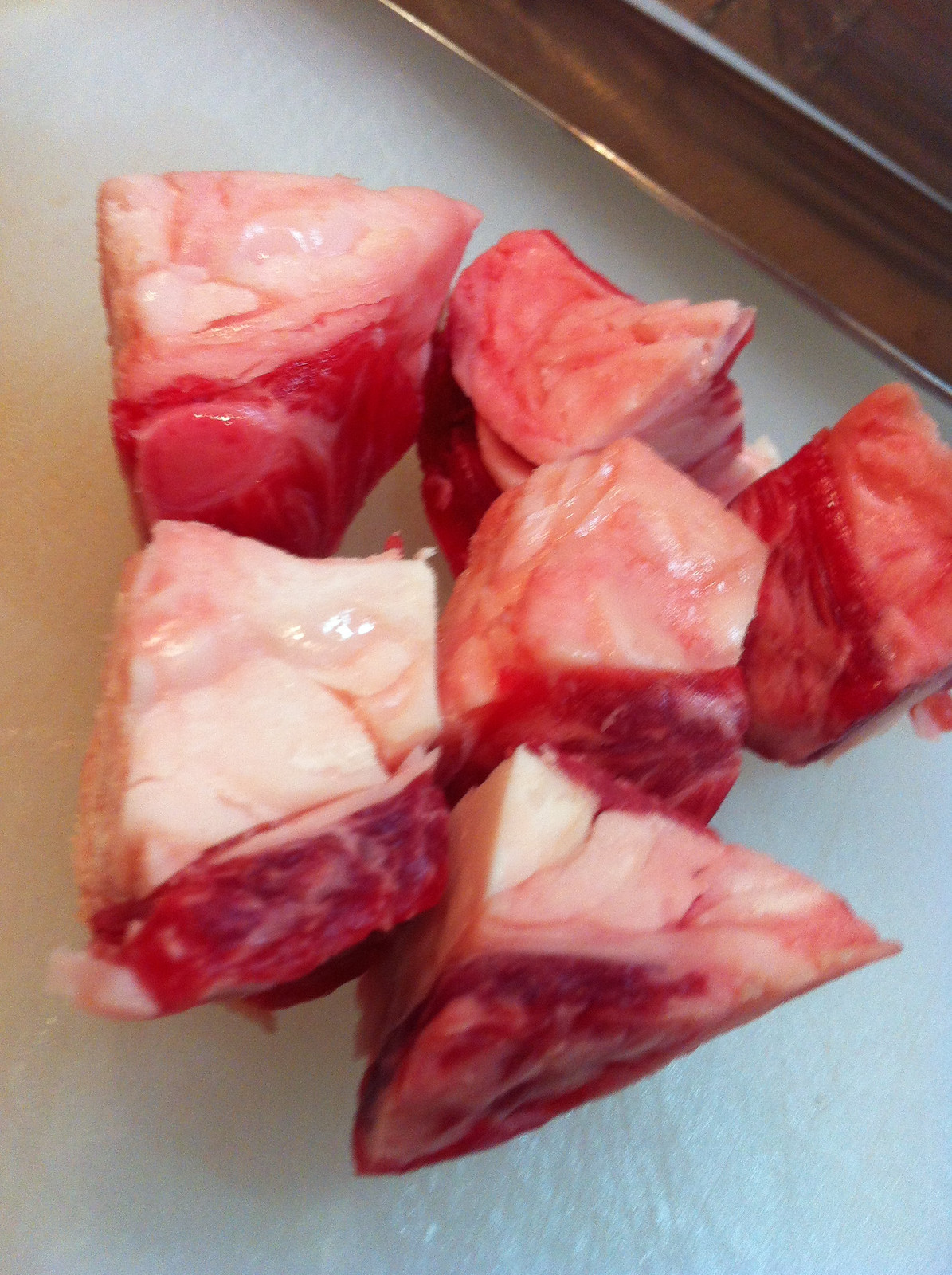This image features a variety of raw meat cut into small, bite-sized cutlets that resemble cubes or triangles. The cutlets appear to be from steak or possibly lamb, characterized by a layer of fat and a slightly bloody appearance. They are arranged on what seems to be a white table or parchment paper, creating a visually appealing display that looks delicious and ready for cooking. The setting has a fun and relaxed design, enhancing the overall charm of the scene.